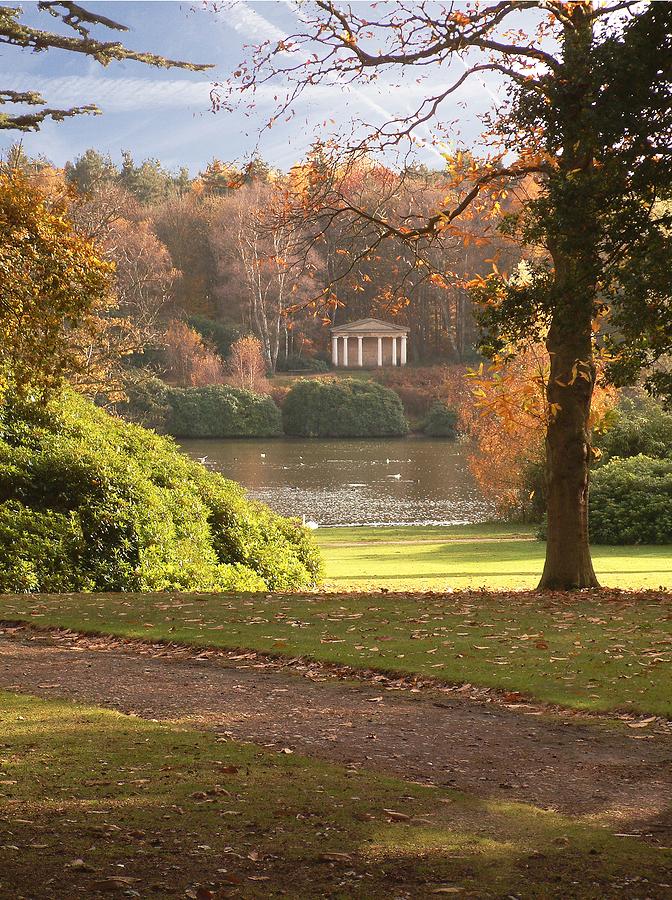This vibrant autumn photograph captures a serene park scene with meticulous details that highlight the interplay of natural elements. In the foreground, a dirt path meanders diagonally from the bottom right to the upper left, surrounded by green grass adorned with scattered brown leaves. To the right stands a thick-trunked tree with a few orange leaves clinging to its spindly branches, while on the left, a green bush and a yellow-leaved tree punctuate the lush landscape.

Beyond the foreground, a silver-gray lake glistens under the subtle blue sky crisscrossed by white airplane trails. Swans gracefully float on the water, with one majestic swan resting on the shoreline. Across the lake, similar green bushes and a small, elegant marble temple-like structure with six white pillars and a brownish-white triangular roof catch the eye. Behind this structure stretches a distant forest, a tapestry of green, leafless, and golden-hued trees that frame the horizon. This detailed composition with its mix of vibrant greenery and autumn colors beautifully captures the essence of an idyllic fall day in the park.